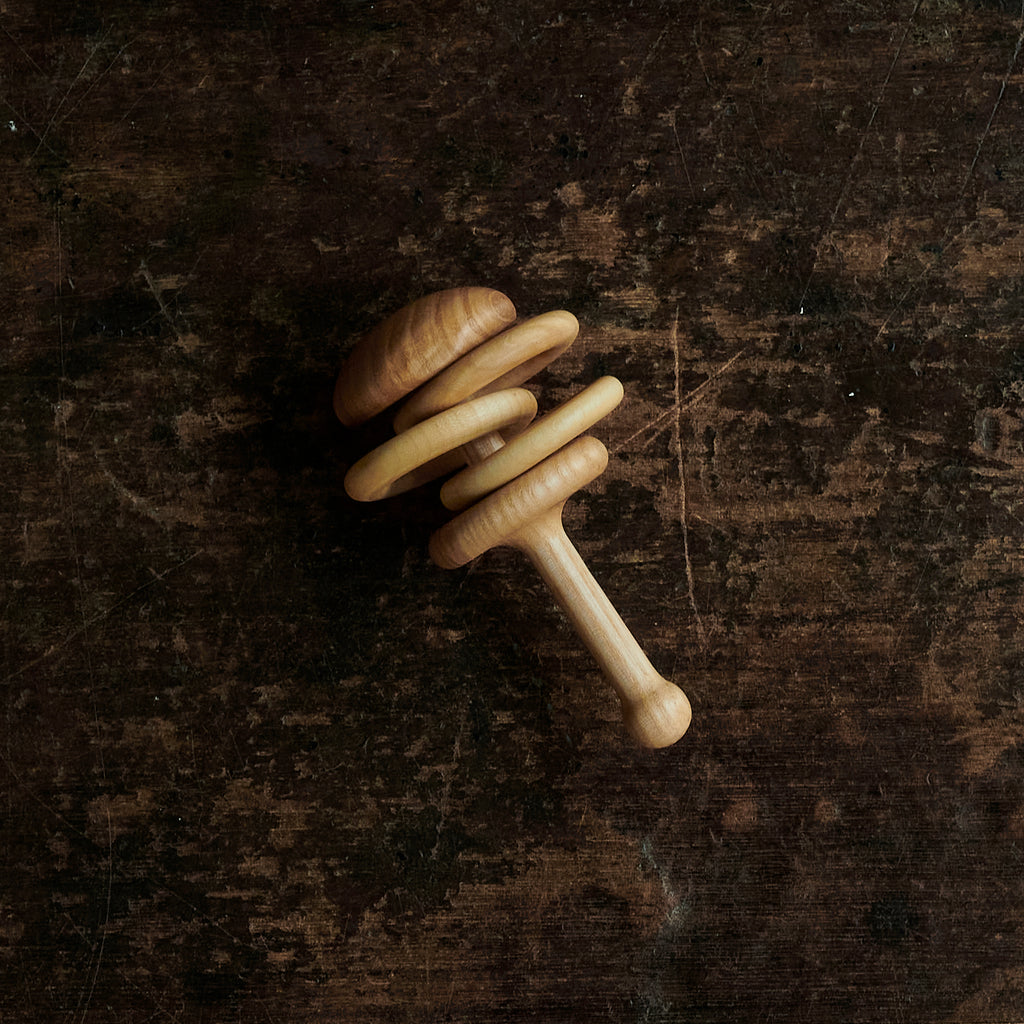The image depicts a finely sanded, intricately carved wooden dowel laying on a dark brown surface that features whitish scratches and carvings. The dowel starts with a circular ball-like knob at the bottom right, transitioning into a handle that can be held. Off to the left, adjacent to the handle, is a round disc, followed by three wooden hoops stacked on the dowel. These hoops are intricately positioned, with one hoop directly attached to the base, another around the pole with a visible gap, and the third closely adjacent to the second. The entire dowel culminates in a rounded, carved wooden top, resembling a bun. The craftsmanship suggests it has been carved from a single piece of wood, indicating no visible joints or connections, and it can be spun around, possibly functioning as a rattle or a noise-making tool.